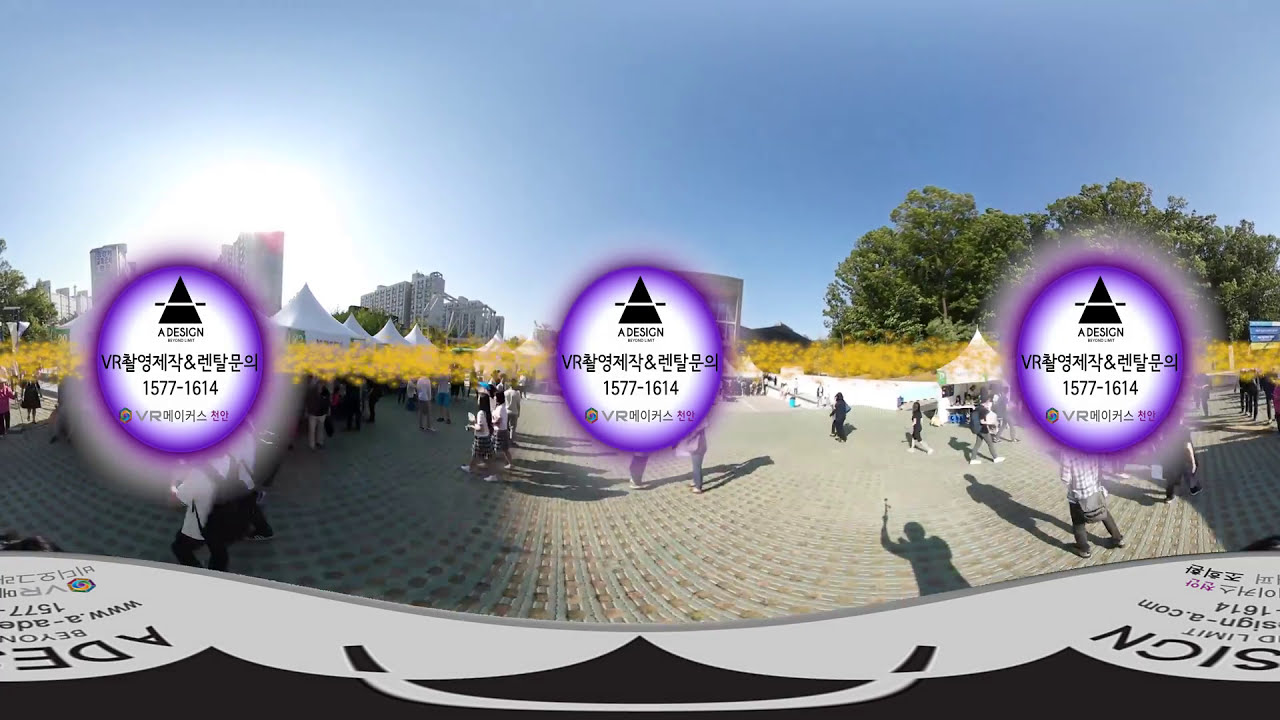This photo, taken outside on a sunny day, captures a lively scene reminiscent of a fair, festival, or open market area. In the background, you can see a vibrant sky, trees, and buildings in the distance, with pavilions and public stands closer to the foreground. People in warm-weather attire are seen meandering through the scene. The image has a 360-degree perspective, offering a broad view of the event.

What stands out, however, are superimposed graphic elements: a fuzzy yellow beam of light stretches across the entire image. Over this beam, there are three identical purple orbs that transition to white towards their centers. Each orb contains text in both English and Chinese (though one account claims it's Korean), stating "A Design VR," followed by the numbers 1577-1614, and followed by more text in the foreign language. There's also a prominent black triangle logo intersected by a line; the line appears white over the triangle and black outside of it. The composite design creates an intriguing overlay to this bustling outdoor scene, adding a layer of digital artistry to the photo's documentation of the day.